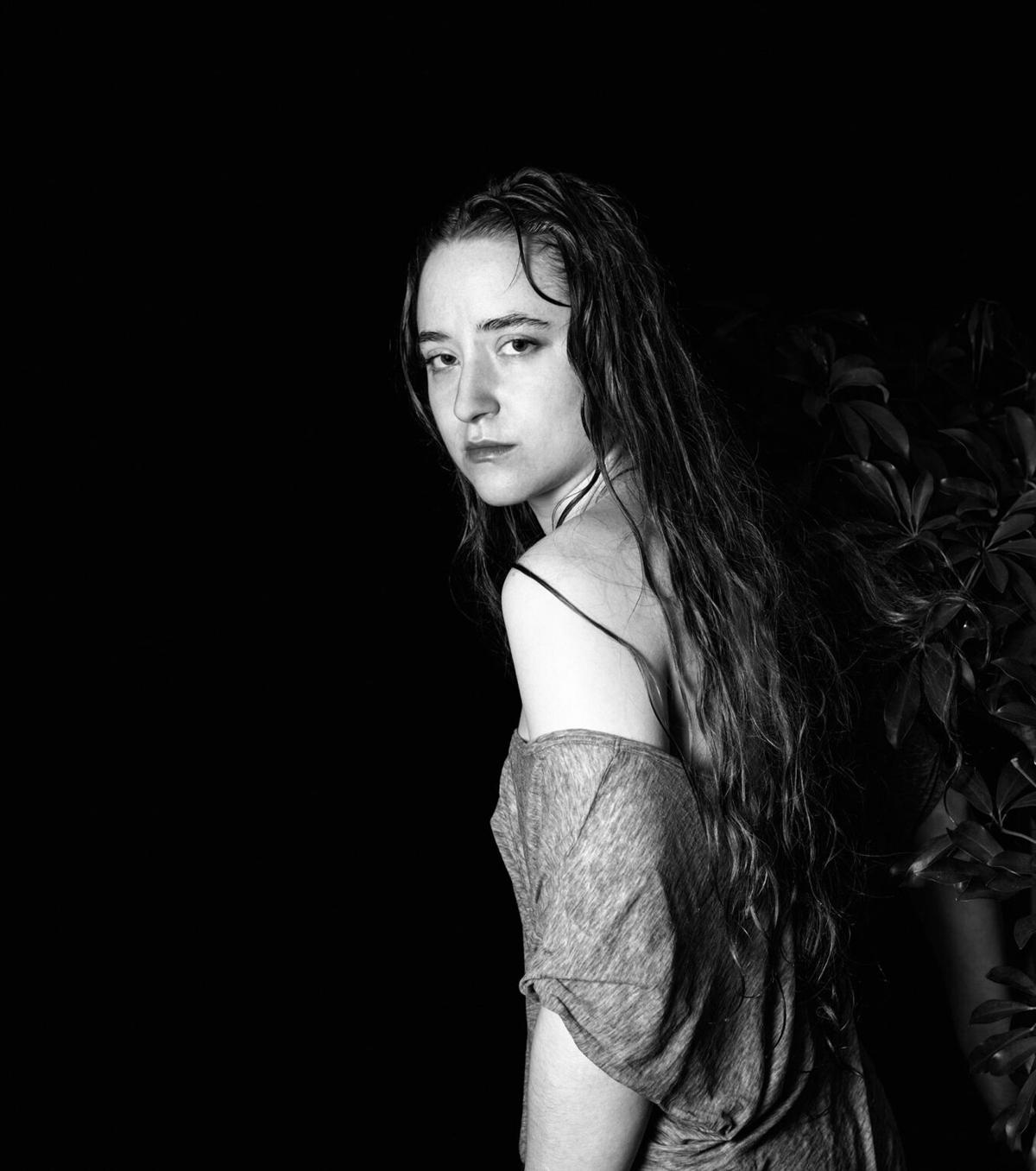In this black-and-white photograph, a Caucasian woman with long, wavy hair that cascades down her back stands out against a very dark background. Her hair appears wet, adding to a serious and somewhat somber expression on her face. She is turning her head toward the viewer, although her body is angled to the left side of the image, creating an impression of a no-nonsense demeanor. The photograph is cut off around her waist, showing that she is wearing a cotton cover-up or long shirt, draped over her arms. A tall tree is visible in the lower right part of the picture, reaching approximately her height. This image, evocative of a modeling shoot, captures a moment that blends poise with a hint of melancholy.